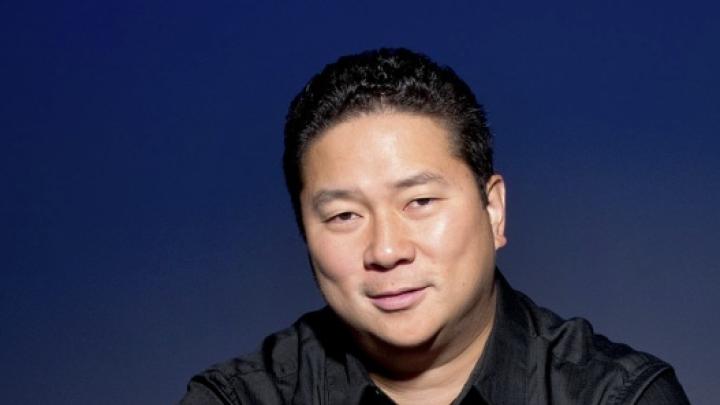This image showcases an Asian man with short, black hair combed back from his forehead, standing out against a navy blue background. The man, centered in the frame and occupying the entire image, exudes a somewhat confused yet smiling expression. His face features light skin, brown slanted eyes, and a wide but thin-looking nose. A shadow of a mustache is visible over his top lip, and his slightly open mouth reveals dimples in his cheeks. He is dressed in a black collared shirt, possibly made of polyester, and there's a faint shadow under his chin. The background is plain, uncluttered, and navy blue, providing no additional context to the scene.